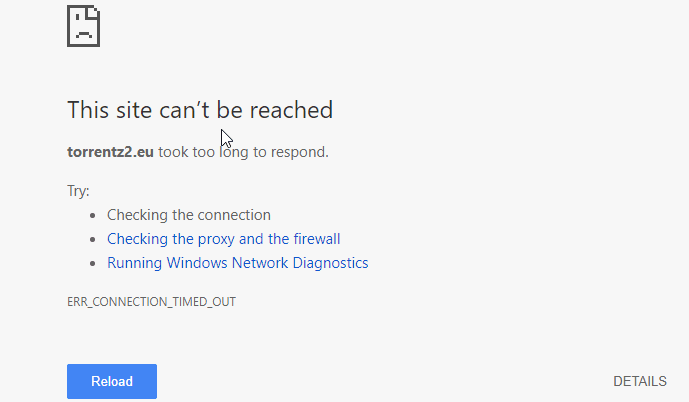Screenshot of a Google Chrome browser displaying an error message. At the center of the screen is an icon of a page with a frowny face, accompanied by the text: "This site can't be reached. Torrentz2.eu took too long to respond." Beneath the main message, it suggests troubleshooting options, including "Try checking the connection, checking the proxy and the firewall, running Windows Network Diagnostics." The error code displayed is "ERR_CONNECTION_TIMED_OUT". The interface includes a "Reload" button and a "Details" link. This screenshot indicates that the Torrentz2.eu site is currently inaccessible, possibly due to maintenance, it being taken down, or other connectivity issues.